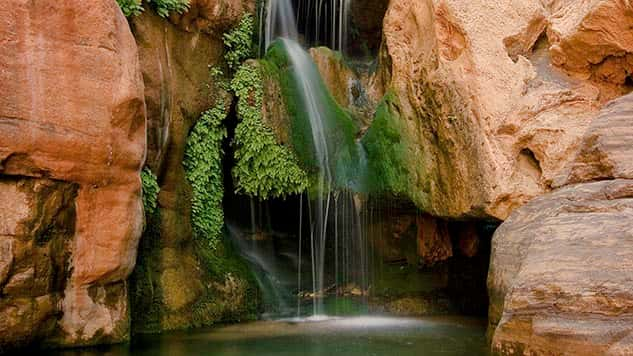This is a serene nature landscape featuring a small, cascading waterfall set amid reddish, clay-colored rocks with brownish striations. The waterfall, composed of multiple gentle streams rather than a high-volume flow, tumbles down the center of the image. This flow nurtures the growth of bright green moss where the water meets the rock surface, giving the middle of the waterfall a vibrant green hue. To the left, on the more moist yet indirectly exposed rocks, various leafy green plants thrive. The waterfall flows into a small, tranquil pool or lagoon at the bottom, possibly leading to an unseen drain. The scene hints at a cool, comfortable cavernous area beneath the waterfall, suggesting a retreat from what appears to be a surrounding desert-like environment. The overall atmosphere is calm and inviting, making it a perfect spot for relaxation.